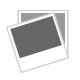The image showcases an old-school PC game, Star Wars Jedi Knight, displayed professionally on a pristine white surface. The jewel case is splayed open, revealing its three-part structure designed to hold two discs. Both discs are positioned side by side in the foreground. Disc one features an angry-faced character wearing a white shirt and sporting short black hair. Disc two depicts a humanoid alien with a blue shirt and a distinctively shaped cone head, appearing to be growling. The case, lacking its original front insert, displays the back cover in the setup, with a description of the game visible but unreadable due to the image's low resolution. The clear cover of the jewel case is to the right, and everything is meticulously placed for a professional photograph, possibly intended for a seller on platforms like eBay.